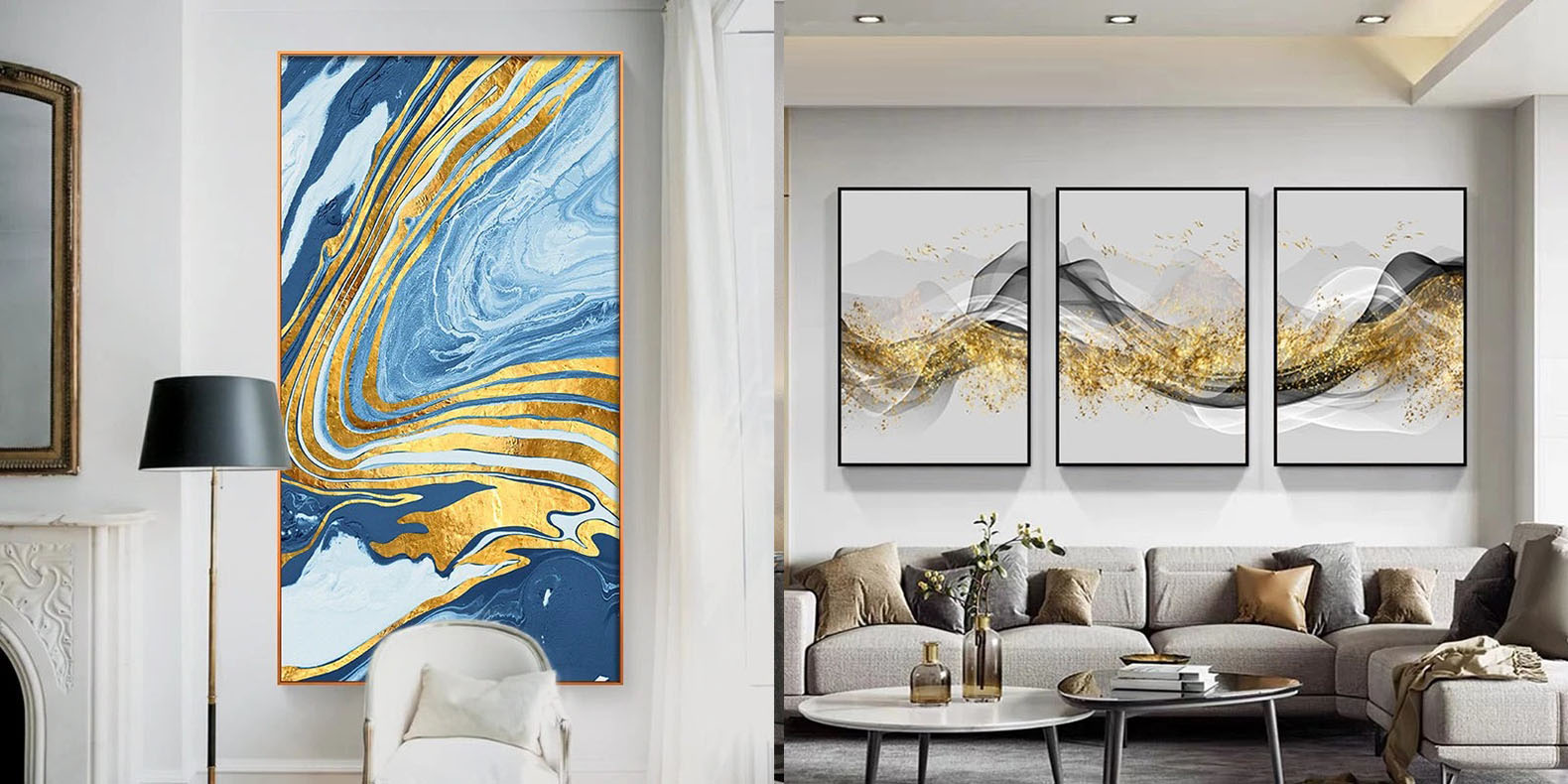This photograph showcases a modern and elegantly decorated interior of a home, featuring a sophisticated living space with detailed decor. Dominating the right side of the room, an L-shaped sectional couch in shades of gray and white is adorned with an array of brown, copper, and gray pillows, and is complemented by a cozy throw blanket. In front of the couch, two coffee tables—one white marble and the other black glass—serve as versatile centerpieces; the black glass table hosts a collection of books, while the white marble one is decorated with stylish, black translucent vases holding vibrant flowers.

On the back wall behind the sectional, a striking triptych piece of wall art captures attention. This three-panel composition features a harmonious black and white line work wave, accentuated with flecks of gold that ripple across the entire piece. The art seamlessly combines into one continuous image despite the division across three canvases.

To the left of this main living area, the image offers a glimpse of a separate corner. Here, a white chair sits invitingly beneath another piece of dramatic wall art. This second artwork, set within a gold-bordered frame, revels in abstract swirls of blue and gold, imbuing the space with a serene, fluid aesthetic. Partially visible are a black shaded, standing floor lamp, a section of a mantelpiece hinting at the presence of a fireplace, and the edge of an elegantly framed mirror.

Overall, the room is a pristine example of contemporary interior design, with its careful coordination of colors and textures, rendering it a tranquil and aesthetically pleasing sanctuary.